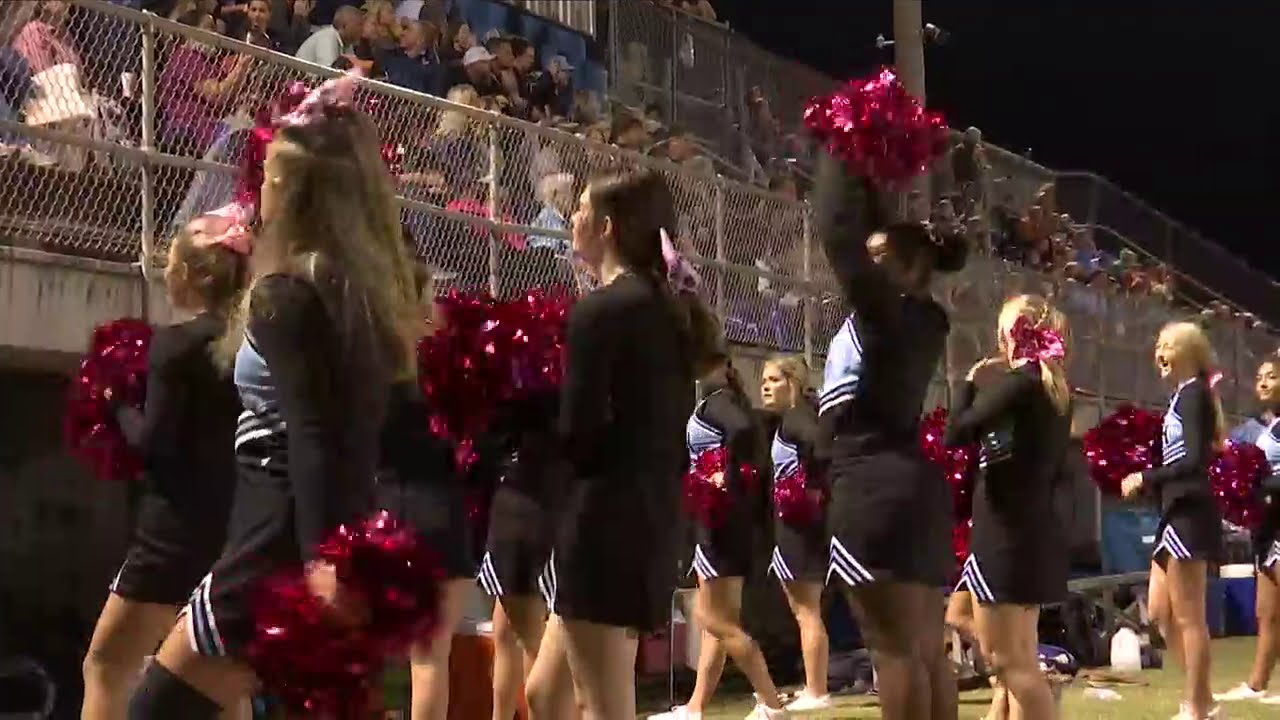In this detailed image, a group of cheerleaders in striking black uniforms with distinctive white stripes along the bottom and across the chest stand in formation facing a crowded stadium. Their outfits are complemented by red pom-poms, which some hold high above their heads while others rest by their sides. Notably, in the center-right, a black cheerleader with her hair styled in an elegant bun holds her pom-poms aloft. Their coordinated appearance is further accentuated by red ribbons adorning their pulled-back hair. The cheerleaders stand on a grassy platform, separated from the enthusiastic fans in the stands by a chain-link fence. A tall pole with lights rises just off-center to the right, illuminating the night sky, which forms a completely black backdrop. The photo, taken horizontally, captures the energy and anticipation of a high school sporting event, framed by small but vibrant stadium seating.